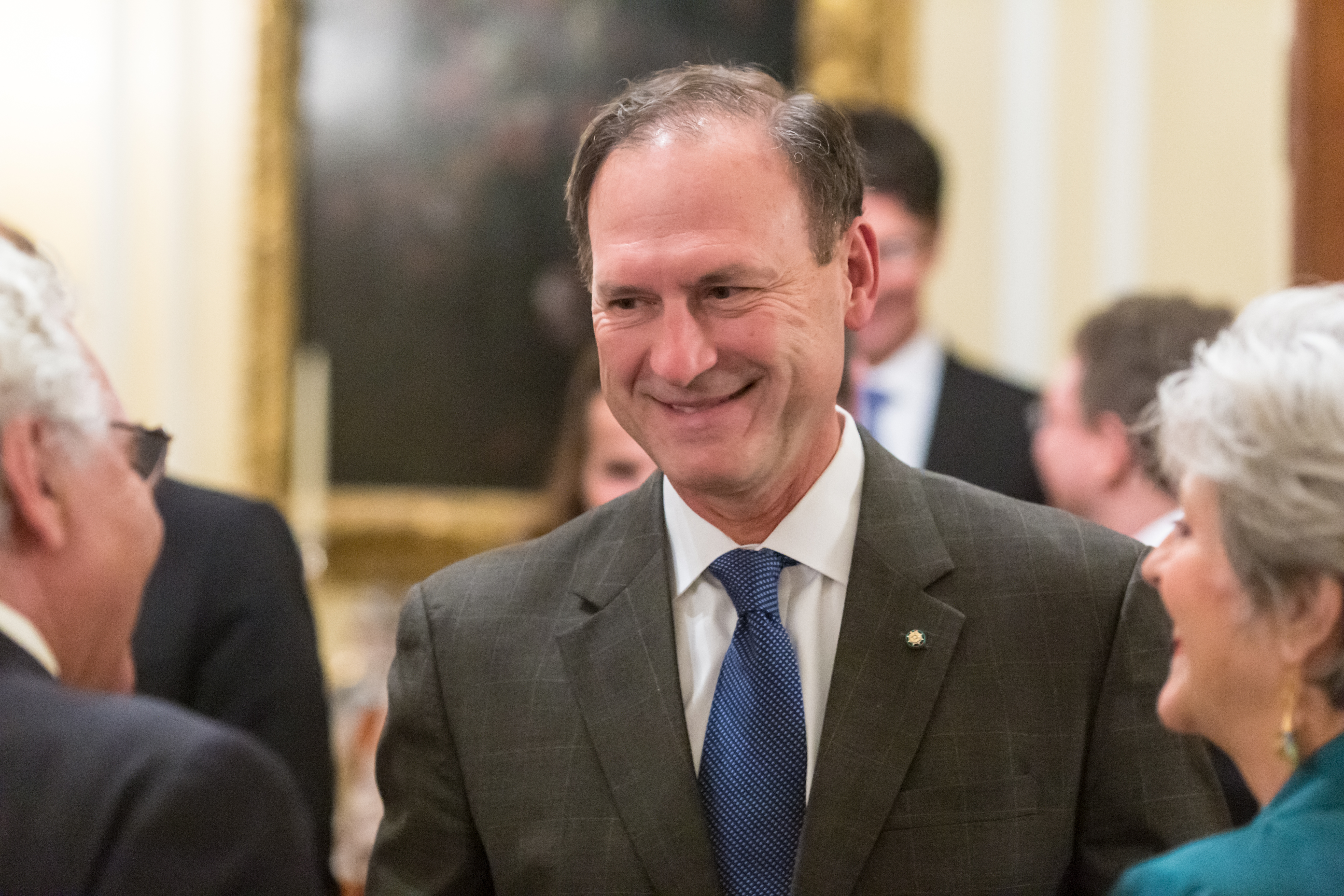In the photograph, a white man, possibly a politician frequently seen on the news, is engaging with a group of people. He is dressed formally in a dark gray suit, a white collared shirt, and a blue tie, and he has brown hair. Prominently, he wears a small pin on his lapel that is distinct from the usual American flag. He seems to be in conversation, possibly shaking hands, with a black man who has white hair. To his left, a woman in a teal suit jacket with graying and white hair stands smiling. The group of individuals he is interacting with appears to be senior in age. In the background, there is a framed artwork with a thick, ornate gold frame, adding a distinguished ambiance to the setting.